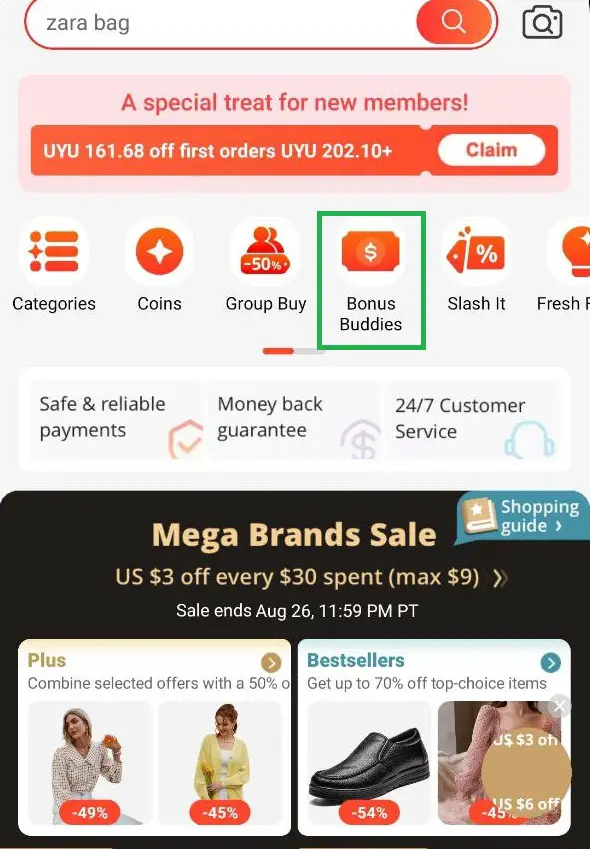This image showcases a promotional offer from Zara for new members. The central element is a shopping bag emblazoned with "Zara" and text highlighting the special treat for new members. Offering significant discounts, the promotion specifies "UYU 161.68 off first orders" and "UYU 202.10 plus." A prominent white button labeled "Claim" encourages users to redeem the offer.

Further down, the interface lists categories such as "Coins," "Group Buy," "Bonus Buddies," "Slash It," and "Fresh." Additional assurances include "Safe and Reliable Payments," "Money Back Guarantee," and "24/7 Customer Service."

A curved black rectangle denotes another offer, stating "Shopping Guide" with details "US $3 off every $30 spent," capping at $9, and "Sale ends August 26, 11:59 PT." At the bottom, more deals are described, such as combining selected offers for a 50% discount and attaining "up to 70% off" on top-choice items.